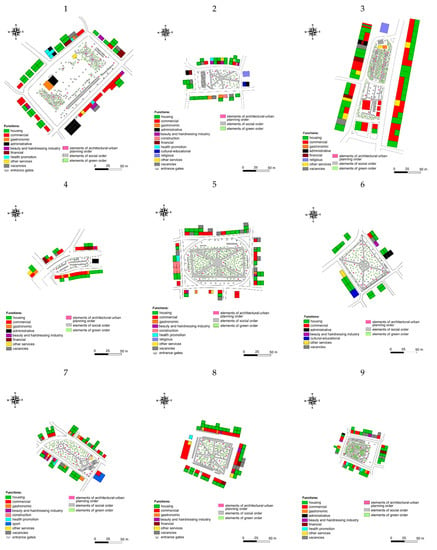The image features nine individual, subtitled diagrams resembling layouts of buildings or parks, organized in a grid of three rows and three columns. Each diagram is detailed with color-coded keys using green, red, orange, black, blue, and yellow, providing a legend for the different areas depicted. These plans, appearing small and intricate, include a compass on the upper left corner and a scaled map distance indicator on the lower right. Despite the overall small size and faint detailing in grey, each plan clearly identifies various sections via the color-coded keys on a white background.